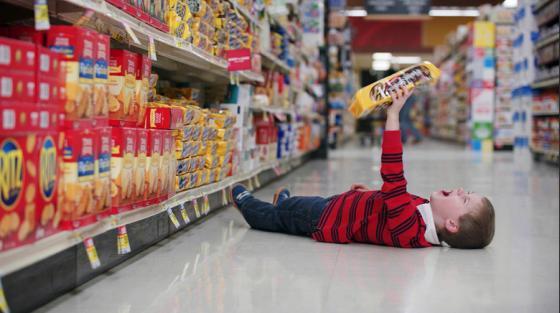This image captures a dramatic moment in a grocery store aisle, depicting a toddler, approximately 1 to 2 years old, lying flat on a glossy white floor, crying. The child, with medium-length brown hair, is dressed in a red and black striped long-sleeve shirt, blue jeans, and matching blue shoes. Clutched in the toddler's left hand, raised towards the ceiling, is a yellow and brown package of Keebler cookies. Surrounding the child on shelving to the left are assorted goods, including Ritz crackers and various other types of cookies and crackers. The perspective of the shot is at floor level, adding to the intense, emotional, and somewhat humorous scene, potentially resembling an advertisement for the cookie brand. Remarkably, the aisle appears devoid of other shoppers, emphasizing the child's tantrum as the focal point of this grocery store tableau.